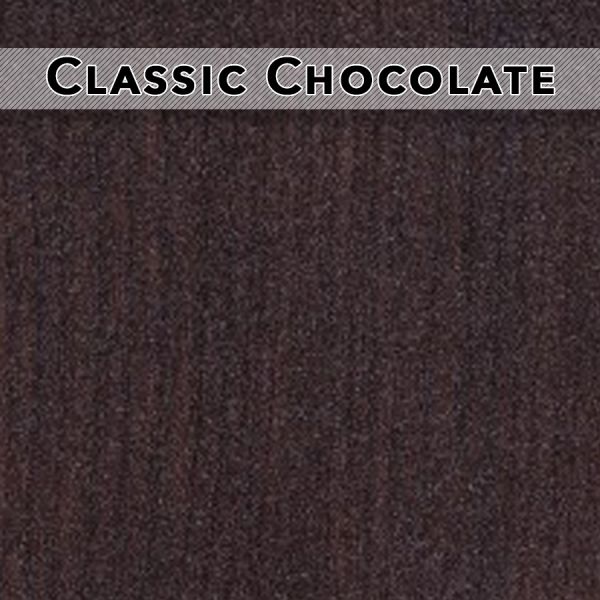The image depicts a square with a predominantly grainy brown background that has a reddish tone, resembling chocolate or possibly fabric due to its texture. Dominating the upper 10% of the image is a horizontally oriented, off-white rectangular ribbon featuring a series of thin, diagonal black lines forming a slash pattern, akin to pinstripes. This ribbon, which spans the entire width at the top, hosts bold black text with a white outline that reads "CLASSIC CHOCOLATE" in all capital letters. Interestingly, the two 'C's at the beginning of each word are slightly larger than the remaining letters, adding emphasis. This simple yet striking design ensures that the phrase "CLASSIC CHOCOLATE" prominently grabs attention.